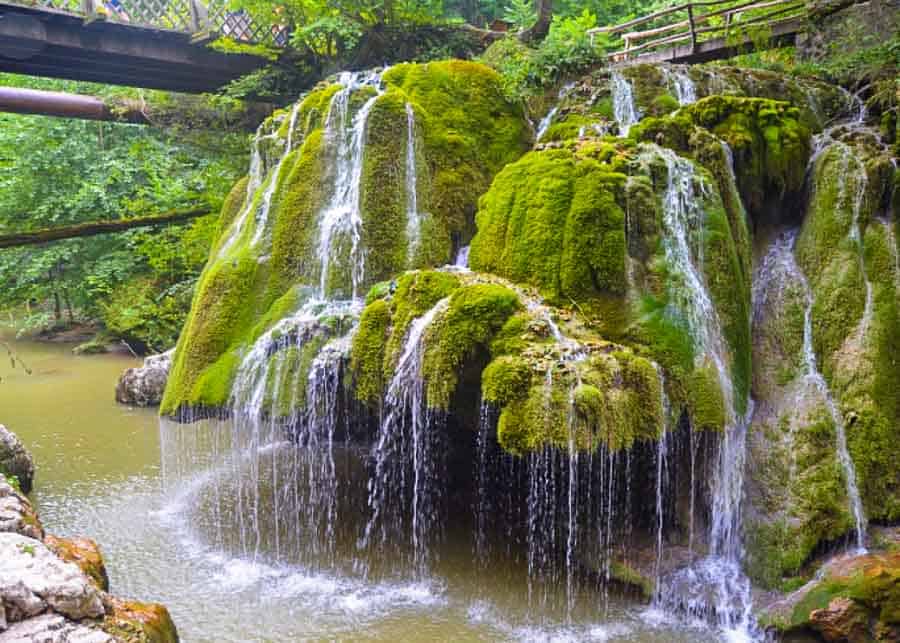The photo captures a serene nature scene outside on a sunny day, featuring a small, unusual waterfall cascading over a moss-covered formation rather than over typical cliffs or rocks. The waterfall appears intermittent, as suggested by the lush green moss covering its path. This green, mossy formation is framed by dense greenery, including bushes and trees. Two unique bridges connect at different angles above the waterfall; one bridge is metallic and the other wooden. Below, a river with murky, greenish-brown water flows, bordered by scattered rocks visible on both the lower left and right sides of the image. The upper part of the picture reveals part of a walking trail with a crosshatch patterned railing on one side of a hill, adding a human element to the scenic view. The colors are vivid, dominated by greens, browns, and whites, enhancing the natural beauty of this rural, wooded area. There are no people, animals, or text visible in this idyllic and peaceful outdoor setting.